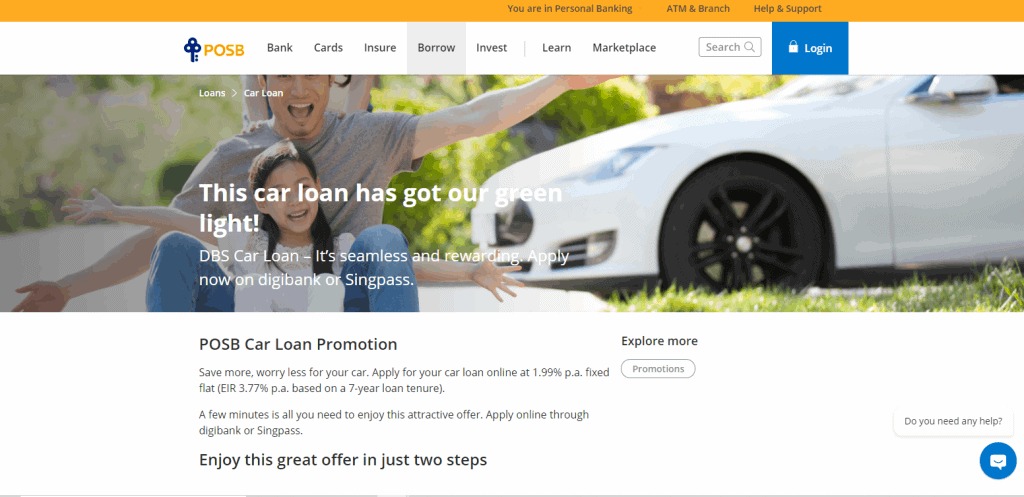**Detailed Caption:**

The image is a landscape screenshot from a website's personal banking section. Spanning from the upper left to the upper right corner, there's a prominent orange stripe. Centered at the top, the text reads "You are in Personal Banking," followed by navigation options: "ATM and Branch" and "Help and Support".

Below the orange stripe, the background shifts to white. This section starts with the POSB logo next to a blue key icon. The navigation menu includes "Bank", "Cards", "Insure", and a highlighted gray tab labeled "Borrow," indicating the current section. Other menu options like "Continue," "Invest," "Learn," and "Marketplace" are also visible. Additionally, there is a search bar and a blue "Login" button that indicates it is secure.

The following row features a large image occupying the majority of the space. In the foreground, a young light-skinned girl sits in front of a man, with a bright white car to their right. Superimposed text reads: "Loans, Car loan. This car loan has got our green light. DBS Car Loan - it's seamless and rewarding. Apply now on Digibank or SingPass."

Further down, a promotional banner for the POSB car loan offers attractive terms: "Save more, worry less for your car. Apply for your car online at 1.99% PA fixed flat. Based on a seven-year loan tenure. A few minutes is all you need to enjoy this attractive offer and apply online through Digibank or SingPass. Enjoy this great offer in just two steps."